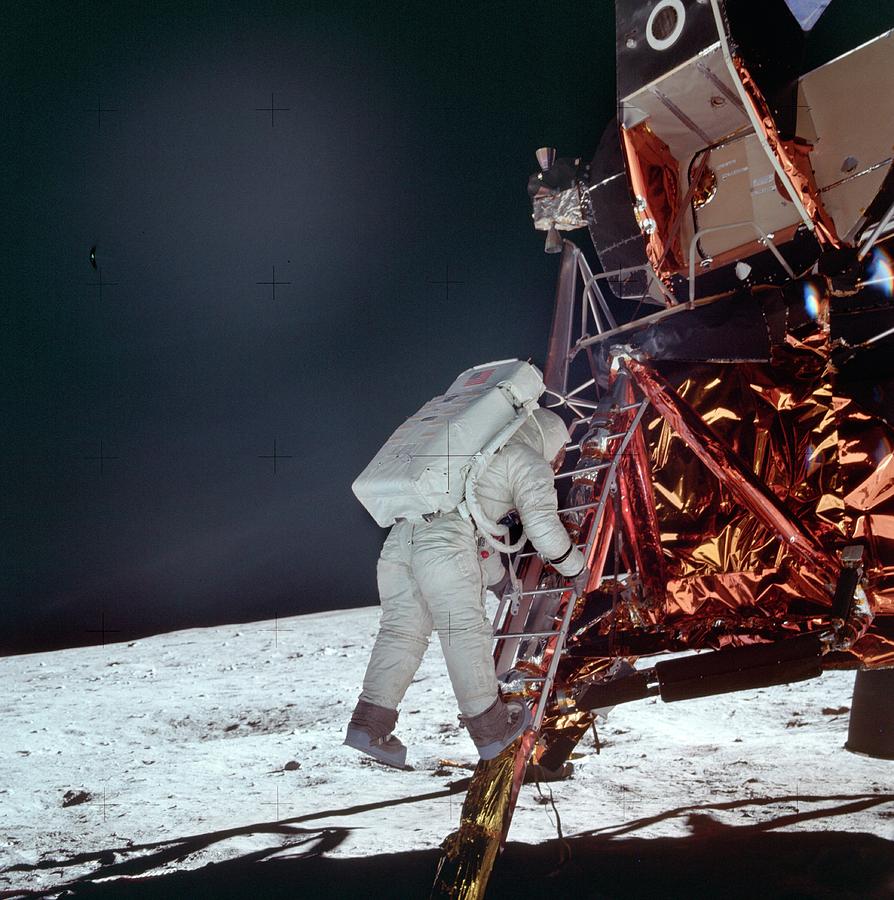In this incredibly detailed photograph of a moon landing, a solitary astronaut in a bulky white suit with a matching backpack adorned with an American flag is captured mid-step on a ladder. The astronaut, facing away from the camera, has both hands and one foot on the ladder while descending from a brightly lit lunar orbiter. The orbiter stands out with its striking hues of orange and gold and is structured with an array of boxes, metal scaffolding, and pipes. A small door at the top of the orbiter indicates where the astronaut emerged. The vast, grayish-white surface of the moon sprawls beneath, marked by craters and illuminated by the orbiter's shadow stretching towards the bottom left corner of the image. The inky blackness of space forms a stark backdrop, and black plus signs dotted across the photograph add to its scientific and historic significance.